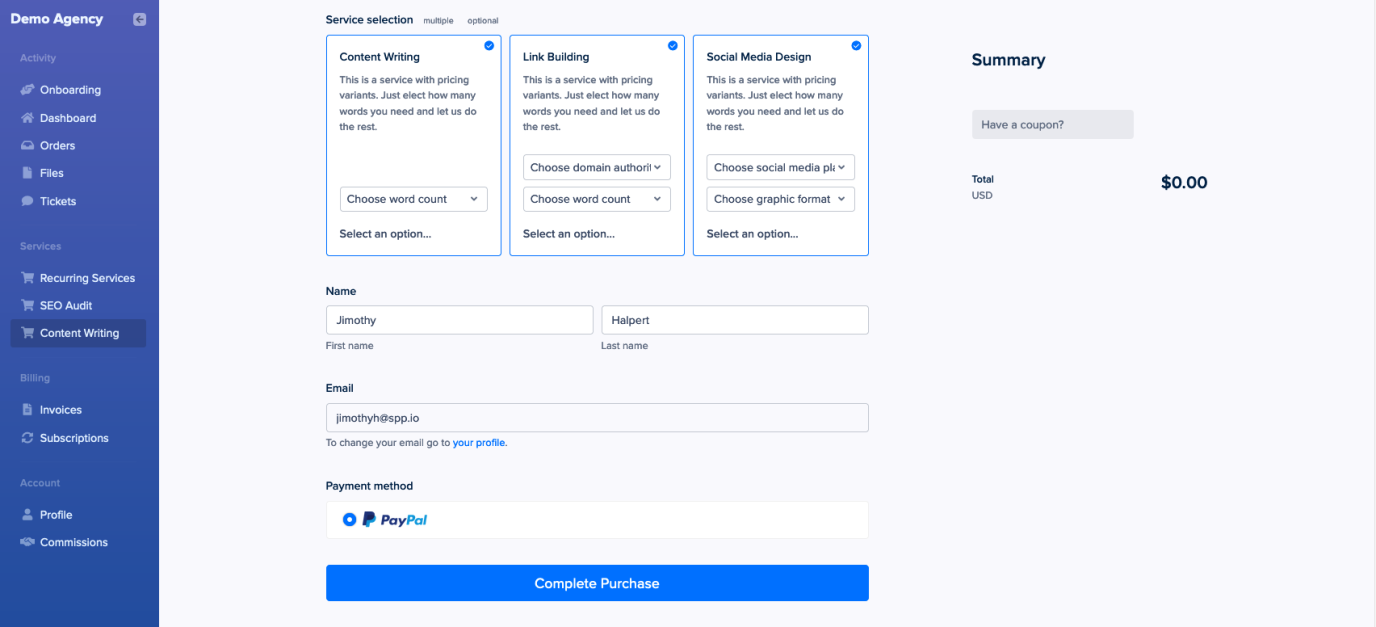On the left-hand side of the image, a blue vertical rectangle lists menu items from top to bottom in white text with certain sections in gray. The top section is labeled "Demo Agency" followed by "Activity" in gray. Below "Activity," in white text, the options are "Onboarding," "Dashboard," "Orders," "Files," and "Tickets." Further down, there's a gray section labeled "Services." Within this section, it lists "Recurring Services," "SEO Audit," and "Content Writing." Moving lower in another gray segment labeled "Billing," this section includes "Invoices" and "Subscriptions." Further down, there is a gray section labeled "Account," comprising "Profile" and "Commissions."

To the right side of this menu, the page is labeled "Service Selection," prominently displayed at the top. Below this heading, there are three rectangular boxes labeled as follows: the first box says "Content Writing," the second box says "Link Building," and the third box says "Social Media Design." Below these three selection boxes, there is a line labeled "Name."